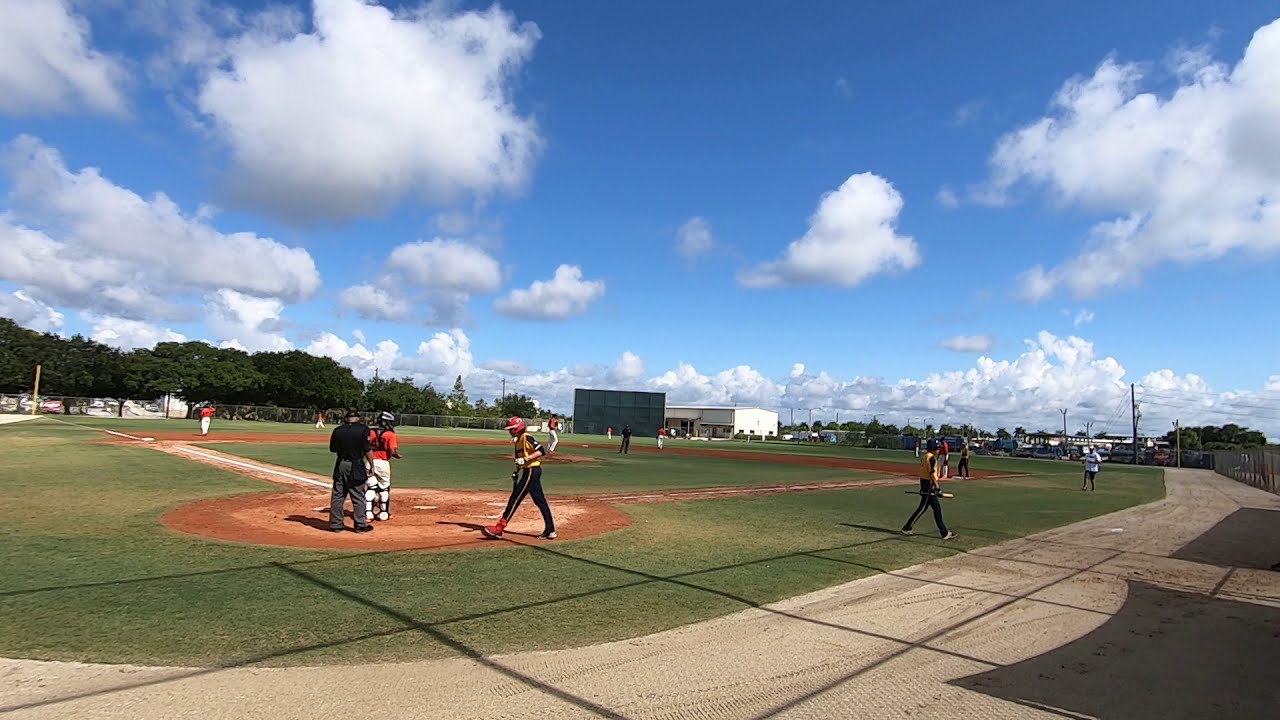In this vibrant image of a baseball game, taken from behind home plate, the scene captures a lively and sunny day under a mostly blue sky adorned with white clouds. Players from two teams, one dressed in yellow shirts with black pants and the other in red shirts with white pants, are scattered around the field. At home plate, an umpire clad in black and gray stands behind the catcher, who appears to be in red and white. A batter, wearing a helmet, approaches the plate, while another player walks away towards the dugout, bat in hand, likely having just struck out. In the background, a scoreboard is visible amidst the green trees that trace the perimeter of the field, which is enclosed by a fence. Beyond the outfield fence, there's a large white building and several smaller structures accompanied by light poles, contributing to the picturesque setting of this quintessential baseball game.